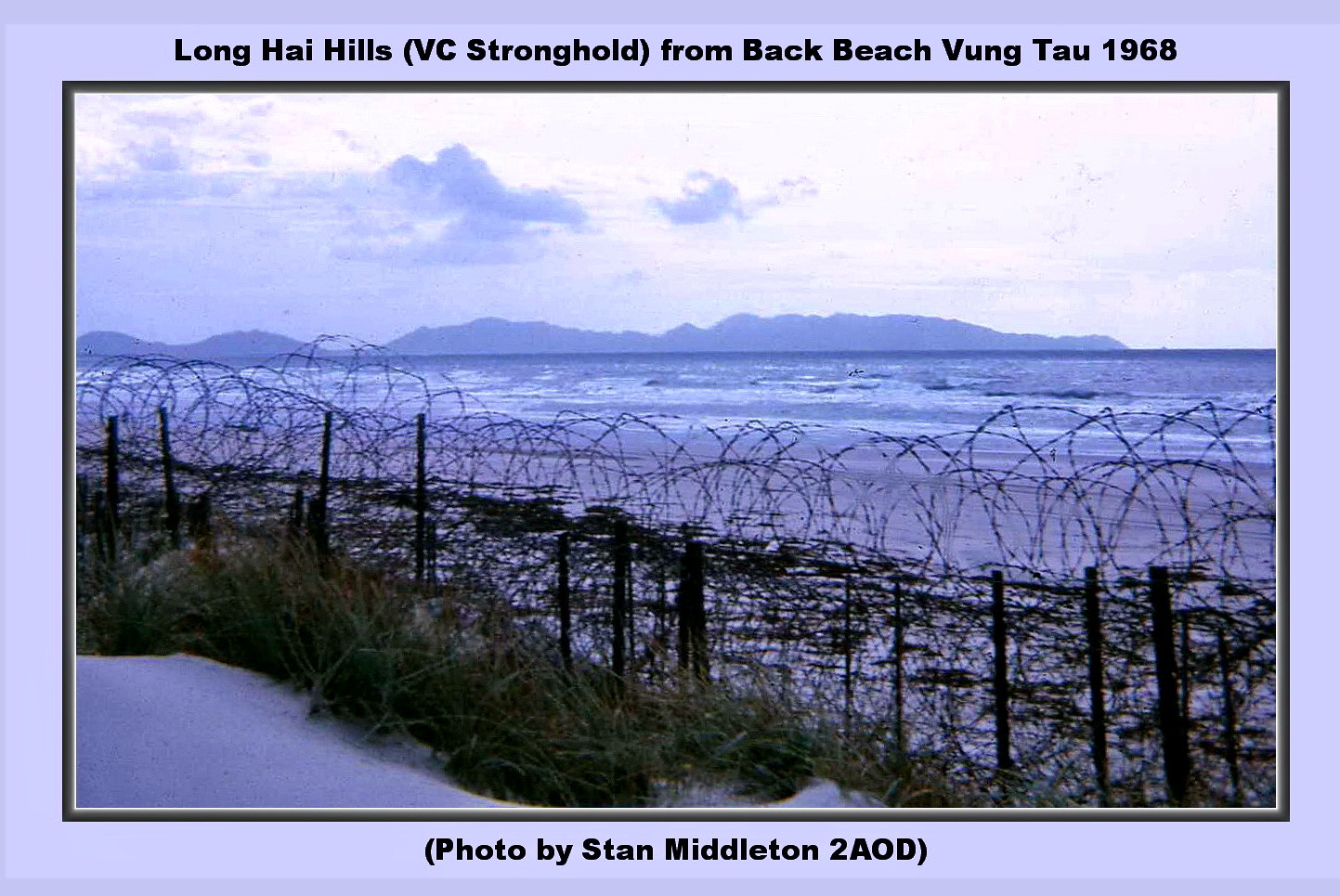The image, enveloped by a striking purple border with an inner black trim, features a haunting scene bathed in a purple tint. Across the top of the purple border, in stark black text, it reads "Long High Heels, VC Stronghold, from Back Beach, Baum-Powell, 1968," while the bottom credits "Photo by Stan Middleton, 2AOD." Dominating the center is a stretch of barbed wire, intricately coiled and supported by sporadically placed posts, looming over patches of green vegetation. Beyond the formidable fence lies a sandy beach with a soft purple hue, where gentle, splashing waves meet the shore. In the background, a distant landscape with rolling hills, some sharply pointed, fades into a sky layered with white and dark purple clouds, contributing to the overall desolate atmosphere.